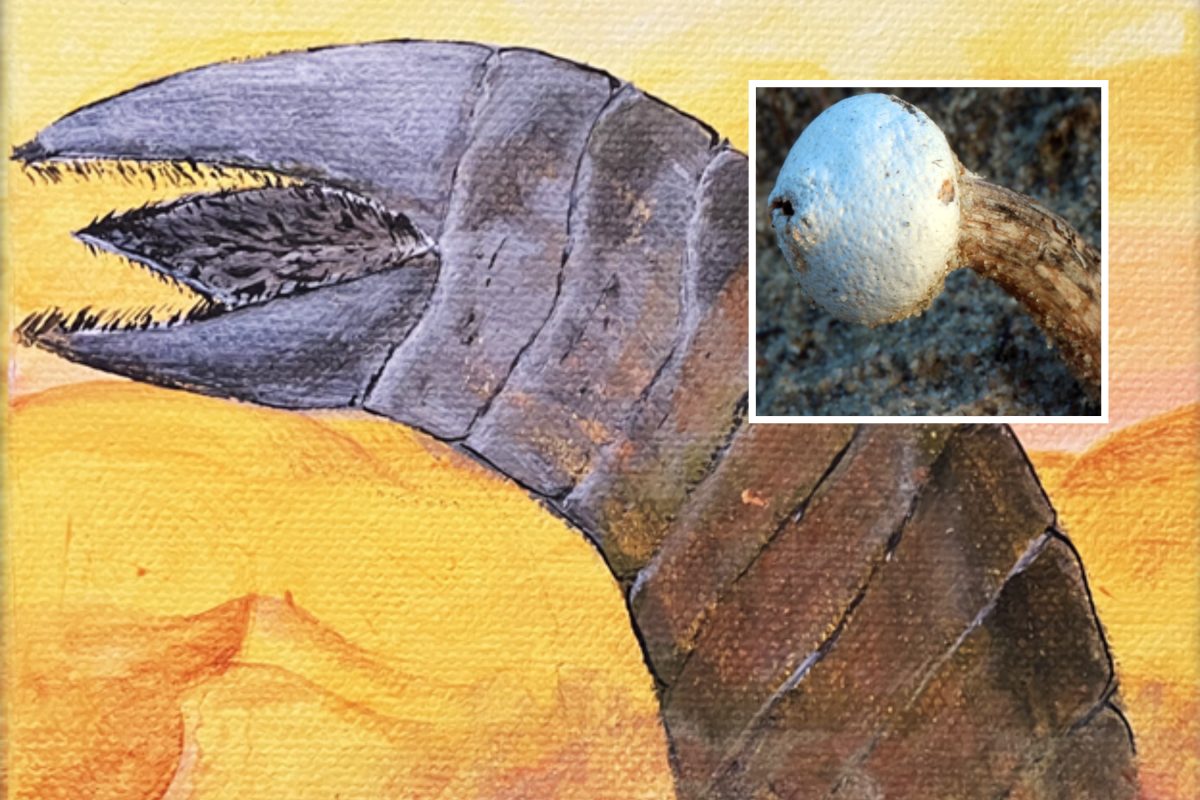The artwork is a detailed, rectangular painting measuring approximately six inches wide and four inches high, set on a textured canvas that enhances its visual depth. The background is rendered in blended tones of yellow and orange, creating a vibrant yet nuanced backdrop with darker orange stripes adding texture, starting from the lower right corner and extending to the upper left. 

Emerging from the lower right corner is a serpentine, tubular creature composed of sequential ringlets that transition from brown to gray as they approach the upper left of the canvas. The creature culminates in a menacing mouth comprised of upper and lower pinchers that resemble a beak, lined with black filament-like teeth. From within this open 'beak' extends a pointed, tongue-like appendage adorned with black stripes.

Overlaying the upper right corner of the painting is a square, color photograph with a narrow white border. This inset photograph appears to depict a real-life counterpart to the creature in the painting. The photo features a textured gray background and shows a similar tubular structure, originating at the lower right and extending to the center. Attached to this structure is a large, spherical white bulb with a small hole on its left side, reminiscent of a type of fungus with a brown stem.